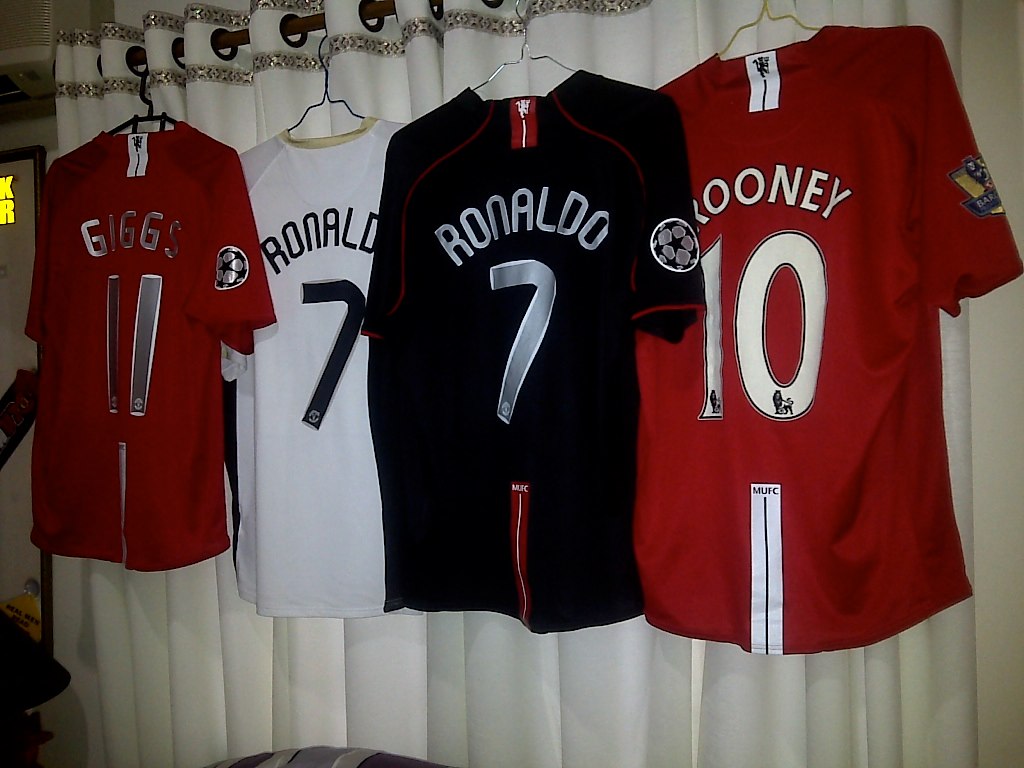This detailed snapshot captures four distinct soccer jerseys, each adorned with recognizable names and numbers, hanging from a white curtain with gold trim and black rings. The first jersey on the left is red with the number 11, albeit the name is not fully visible due to a rumple in the fabric. The next two jerseys both display the name "Ronaldo" and the number 7; they are colored white and black, respectively, featuring silver lettering. The jersey on the far right is red, showcasing the name "Rooney" and the number 10. The curtain rod, in a black or brown hue, supports the curtain, which has a silver lining at the top. The setting suggests a store or a dressing area, evidenced by a partial store sign in the background and a glimpse of a couch at the image's bottom. The jerseys are illuminated by the camera flash, with sunlight streaming in from a window on the left, adding to the ambient lighting.